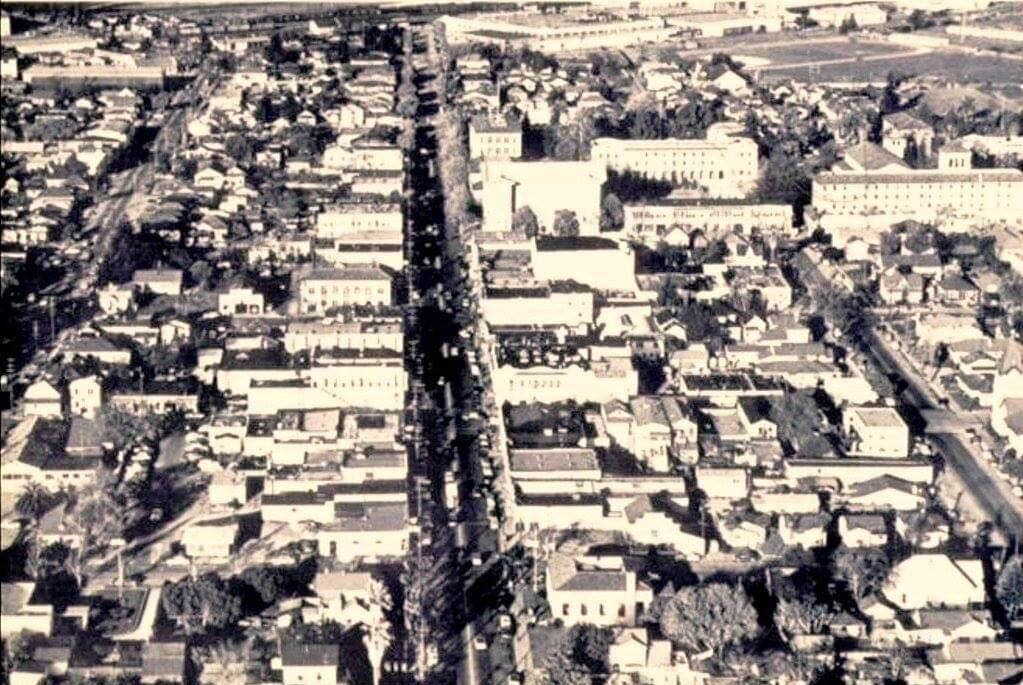This black and white aerial photograph presents a dense, grid-patterned cityscape, captured from a significant height, possibly from a helicopter or airplane, reflecting a vintage era. The image showcases a prominent main boulevard running vertically down the center, flanked by various buildings of different heights and architectural styles. On the left side, there are indications of potential residential buildings, though they are tightly packed, making it difficult to distinguish individual homes. The dominant structures on the right-hand side suggest large factories, office buildings, or possibly government facilities. In the upper right corner, there's a sizable open field, possibly a baseball or sports playing field, adjacent to more large buildings that could be hospitals or university structures. Numerous cars can be seen navigating the streets, contributing to the city's busy atmosphere. The scene embodies photographic realism, capturing the essence of a bustling urban environment from a bygone era.